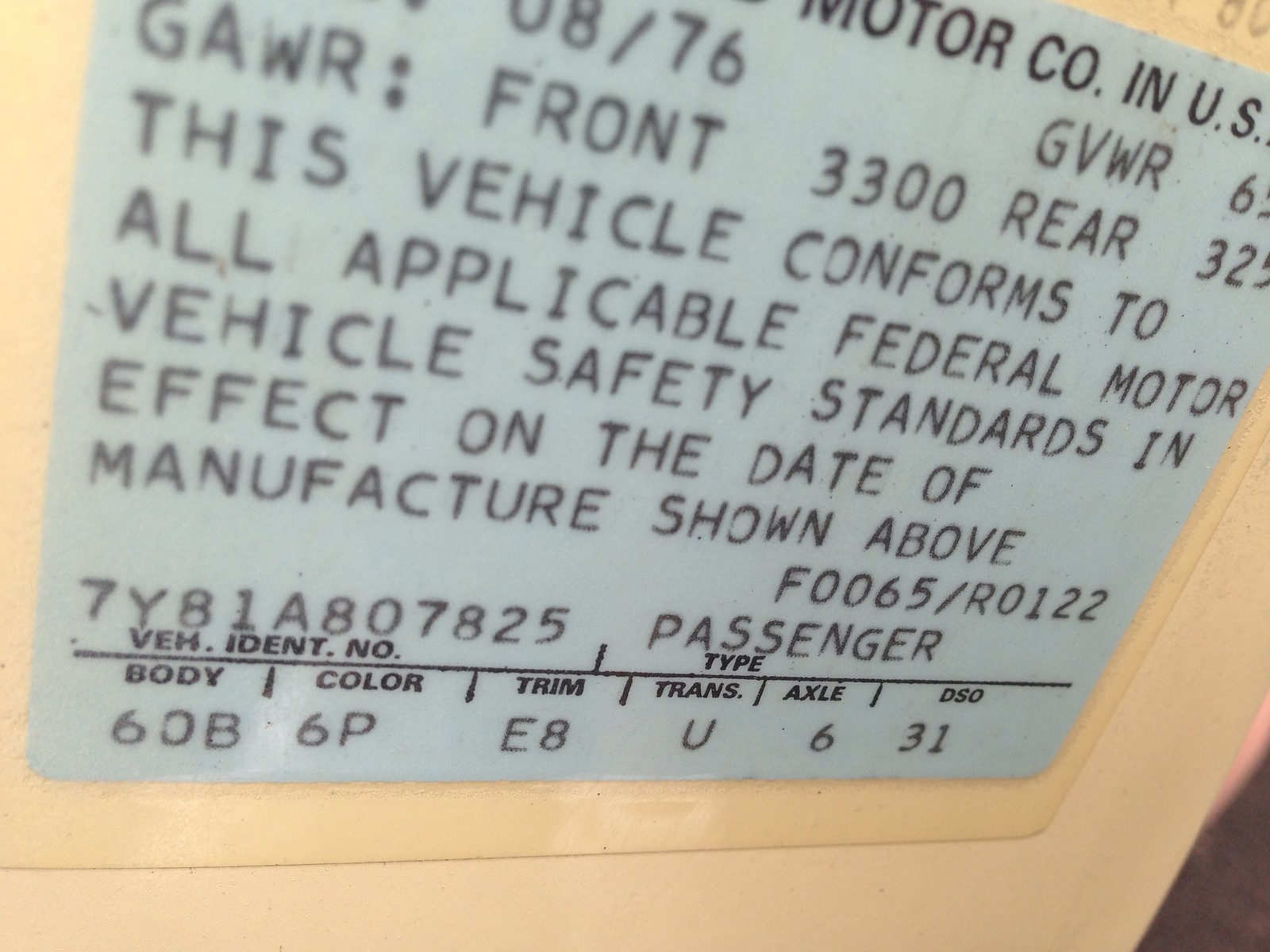The image depicts a close-up of a digital motor vehicle inspection label, slightly rectangular with a light brown frame. The background is light blue or light gray, featuring a considerable amount of black text. The label, which is partially cut off in the photograph, provides essential vehicle details and safety compliance information. Notably, it includes the name "Motor Company USA" at the top and specifies that the vehicle conforms to all applicable Federal Motor Vehicle Safety Standards as of its manufacture date, likely August 1976 (08/76). Further details on the label include the GVWR (Gross Axle Weight Rating) with the front as 3300 and rear partly legible as 325 or 32. It also mentions F0065/R0122, the Vehicle Identification Number (VIN) 7Y81A807825, and identifies the vehicle as a passenger type with the body type 60B. Additional specifications are color code 6P, trim code E8, transmission code U, axle count 6, and DSO code 31. This detailed label serves to validate the vehicle's specifics and compliance with safety standards at the time of manufacture.